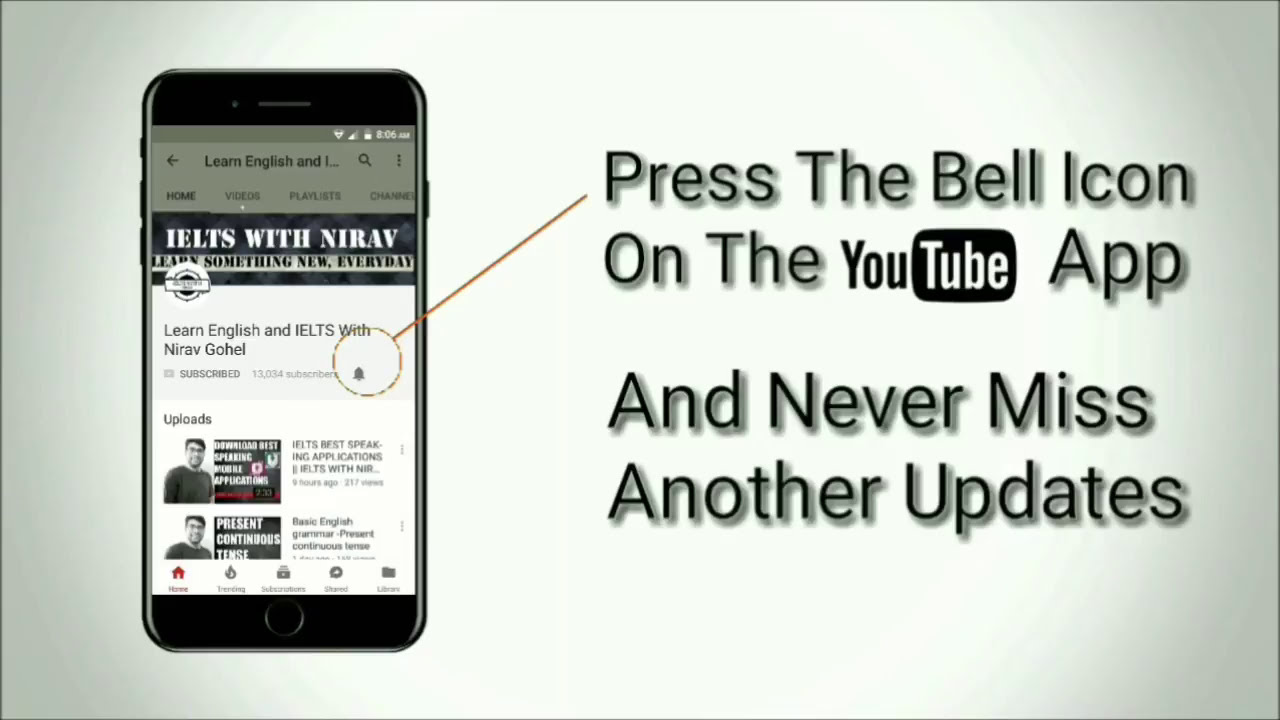The image is a promotional advertisement featuring a black iPhone positioned on the left side of a predominantly green-themed background. The screen of the iPhone displays various texts, including "Learn English and IELTS with Nirav Goel," and highlights different colors such as white, red, and light green. Additionally, the screen shows the YouTube channel's details like uploads and a subscriber count of 13,034, along with a notification bell icon encircled to draw attention. On the right side of the image, there is black text instructing viewers to "Press the bell icon on the YouTube app and never miss another update," though the grammar is slightly incorrect. The overall appearance suggests it is an Indian YouTube channel advertisement aimed at attracting users to subscribe and stay updated with Nirav Goel’s English and IELTS learning content.